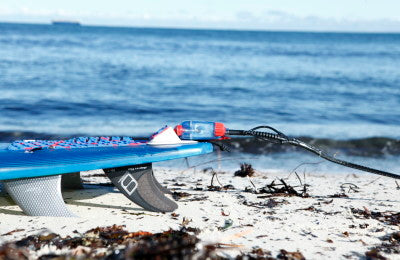The photograph showcases a scenic beach scene under a bright daytime sky with light blue hues and scattered clouds. In the foreground, a vibrant blue surfboard equipped with gray and white fins lies on the pristine, white sandy shore. There’s debris on the sand, including dried seaweed and leaves. The surfboard features a Shark Shield—a shark deterrence device—indicated by an attachment with a black cord. The background captures the vast, blurred blue ocean with visible ripples and waves crashing gently onto the shore. The sun shines brightly, adding a warm glow to the entire scene, with a tiny ship visible on the distant horizon.